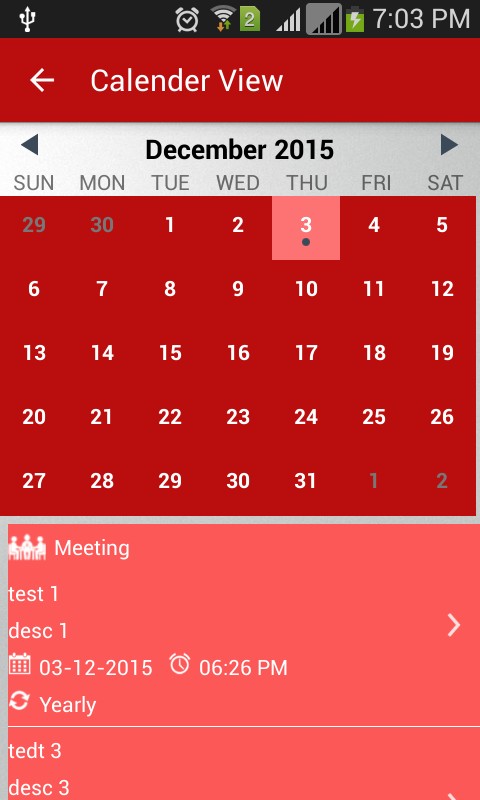This screenshot captures the calendar view of a phone application. At the very top, there's a black status bar displaying standard icons for Wi-Fi strength, battery life, cellular signal strength, and the time which reads 7:03 PM. Additionally, there is a clock symbol, a number 2, and a dog-eared page icon.

Below the status bar, a bright red banner with the text "Calendar View" and a white 'go back' arrow sits prominently. Directly beneath this, the current month and year, "December 2015," are displayed, flanked by black 'go back' and 'go forward' arrows for navigating between months.

The week starts with the days of the week, from Sunday to Saturday, labeled in gray. The calendar grid follows, highlighting the days of December 2015 in bright red, starting with Tuesday the 1st and ending with Thursday the 31st.

At the bottom of the screenshot, an orange-red box appears, signaling an event. This box includes information with icons of people on the left side and the text: "Test 1, Description 1, calendar icon, 3-12-2015."